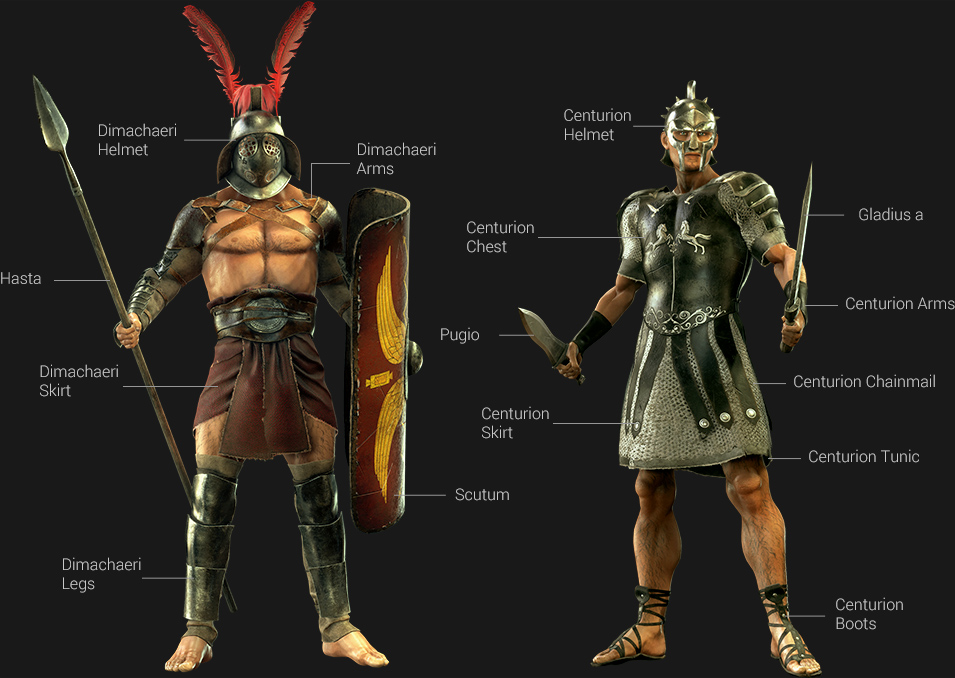In this detailed digital artwork, set against a stark black background, we see two video game-style warrior characters, each meticulously labeled with their gear. On the left is a shirtless warrior adorned with a black or green helmet elaborately decorated with red feathers. His armor includes black knee and shin protectors, a skirt-like fabric, and metallic arm and leg guards. He's armed with a spear and a large, curved red shield labeled "Scutum." His gear is systematically annotated as Demetri Helmet, Demetri Arms, Demetri Skirt, Demetri Legs, and a Scutum. 

To the right stands a fully armored warrior evoking Roman Centurion imagery. This character wears a silver helmet labeled Centurion Helmet, a detailed chest plate labeled Centurion Chest, a corresponding skirt, arms, and boots. He wields a knife and a gladius (short sword). The detailed annotations around him include Centurion Helmet, Centurion Chest, Centurion Skirt, Centurion Arms, Centurion Chainmail, Centurion Tunic, and Centurion Boots. Both warriors exhibit a comprehensive display of labeled equipment, making it clear they are intricately designed characters, likely from a game.